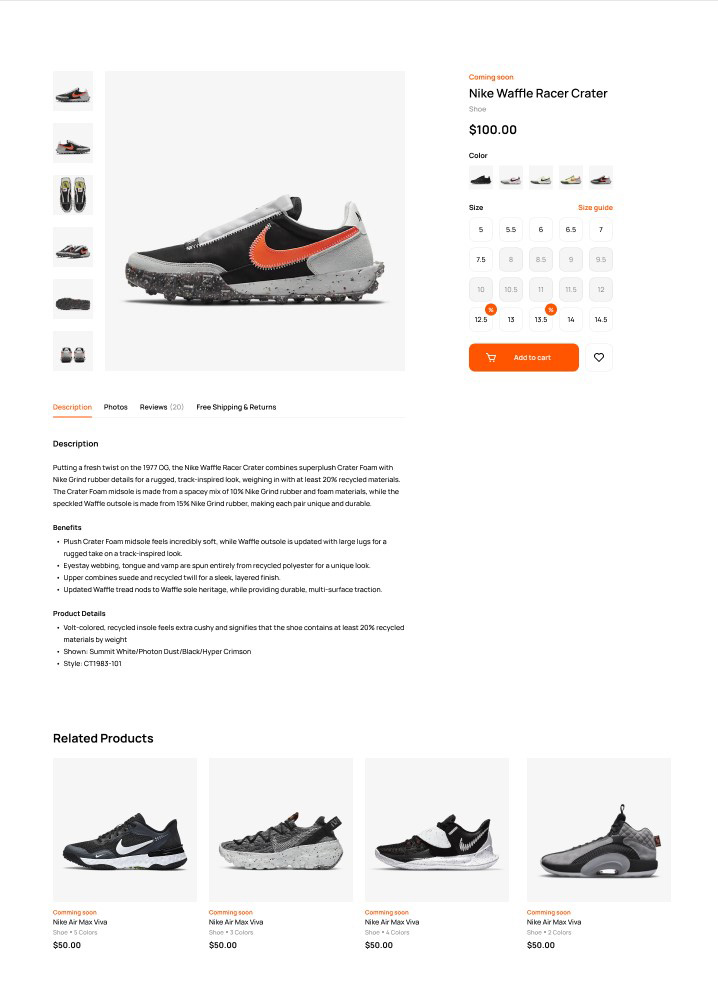Screen capture of a shopping website displaying a product listing. The website showcases the "Nike Waffle Racer Crater" shoe, priced at $100. In the upper right corner, an orange label indicates "Coming Soon" with the product name and price in black beneath it.

On the left side of the screen, a large, detailed image of the Nike Waffle Racer Crater shoe is featured. The black and white sneaker prominently displays a reddish-orange Nike logo. To the left of the main image, there are six thumbnail images allowing users to view the shoe from different angles.

On the right side, beneath the product title, there are options to choose from five different colors. Below the color options, a sizing chart is available, along with a red "Add to Cart" button.

A three-paragraph text description located below the images on the left provides details on the shoe’s description, benefits, and product specifics, though the text is quite small. Further down, a bold heading reads "Related Products." Below this heading, black and white images of four other sneakers are displayed, all identified as "Nike Air Max Vivo" in various styles, each priced at $50.